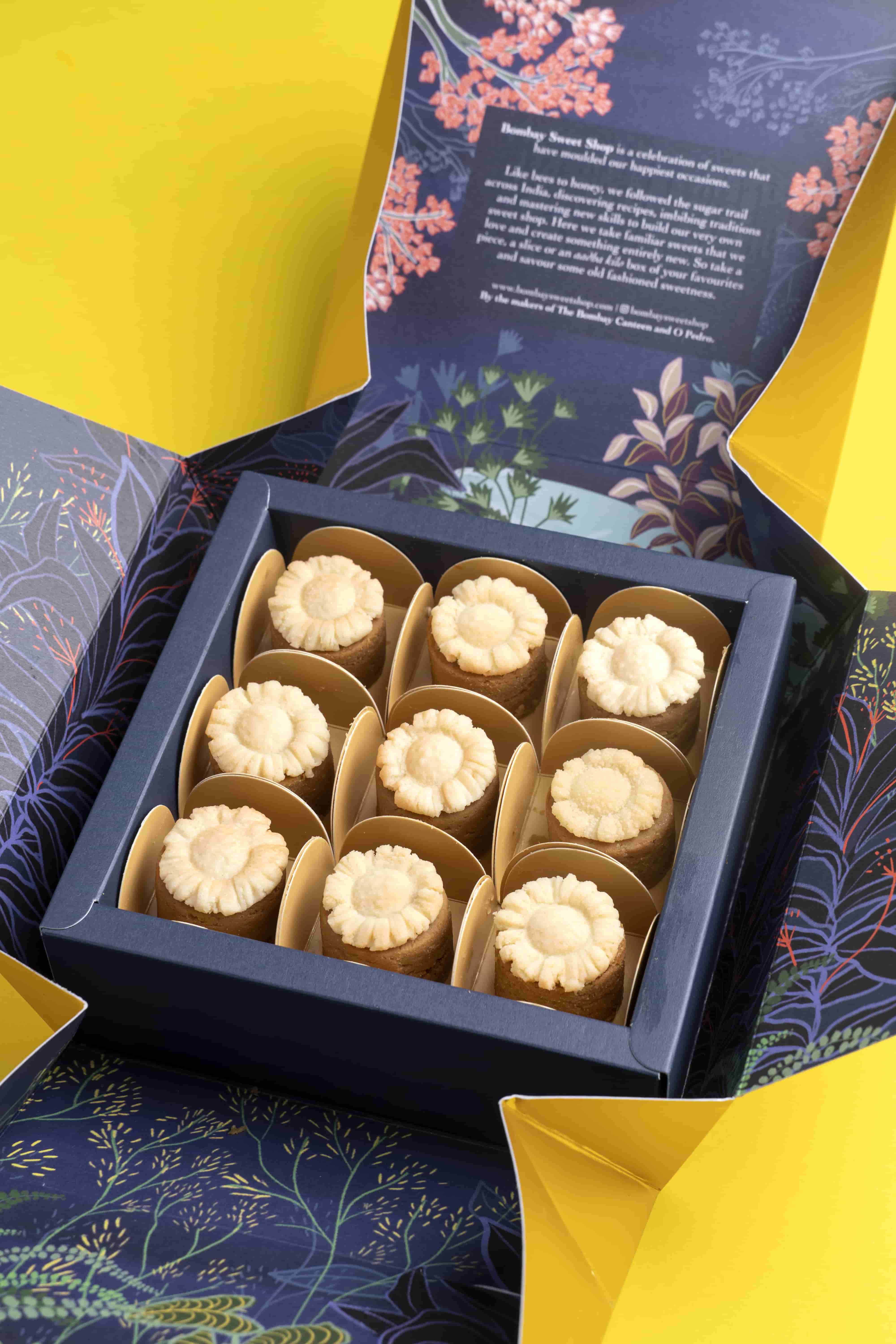This vertical-angle photograph captures an elegant boxed dessert from the Bombay Sweet Shop. The exterior of the box is a simple plain yellow, while the interior unfolds to reveal a stunning floral night scene with blooming trees and plants against a calm navy blue background, evoking a serene "night by the pond" atmosphere. The inside top flap contains some text, although it's challenging to read in the image, but the phrase "Bombay Sweet Shop" is clearly visible, celebrating a tradition of sweets that mark joyous occasions.

Inside, the box meticulously separates nine cylindrical treats, each nestled in its own compartment formed by small brown cardboard dividers. These desserts are medium brown, about an inch in height and slightly wider, and are topped with a delicate, almost white flower shape, adding to their intricate appearance. The overall presentation blends sophistication with an inviting, edible allure, indicating these are possibly small pastries or similar confections rather than fancy soaps. The detailed floral theme and structured organization reflect the high-quality and thoughtful design of the Bombay Sweet Shop's offerings.